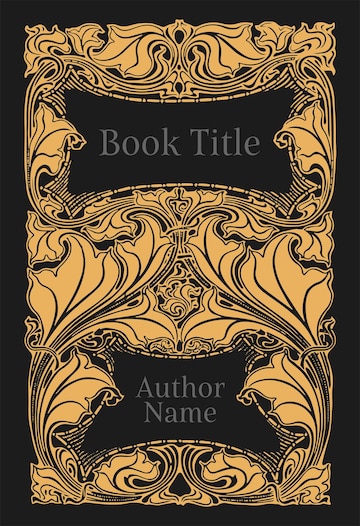The image is a vertical rectangular template for a book cover with a black edge framing the design. Inside, intricate black swirling lines resembling various types of leaves and curves adorn a gold background, creating a mirrored pattern that rises upwards on both sides, forming an elegant symmetry.

At the top, there is a fancier, indented rectangular section also outlined in black with more ornate black lines around the gold. Inside this section, written in gold letters, is the placeholder text "Book Title," indicating where the title of a book would be placed.

Similarly, at the bottom, there is another decorative section with a slightly different, more elaborate shape. This section has a black background and gold lettering that reads "Author Name," serving as a placeholder for the author's name. The entire design maintains a cohesive color scheme of black and gold, lending the cover an exquisite, classic appearance.